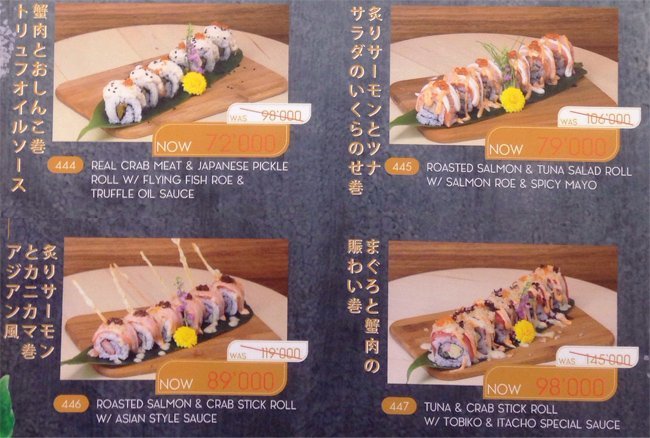The image is a scan of a segment of a sushi restaurant's menu, featuring four different sushi roll dishes, each prominently displayed in one of the four quadrants of the page. Each dish consists of about six slices of sushi neatly aligned in a row and presented on a small brown bamboo serving board, with a leafy green garnish underneath. 

To the left of each sushi image, vertical non-English text, likely Japanese kanji, is presented in a gold color. An orange oval with a white number (ranging from 444 to 447) and the word "NOW" in white uppercase font denotes the current promotion. Each item's old price is shown in white text above the "NOW" oval, with a red, discounted current price below it. The background of the menu features a charcoal gray color that makes the sushi images stand out.

1. **Dish 444**: Labeled "Real Crab Meat and Japanese Pickle Roll with Flying Fish Roe, and Truffle Oil Sauce." It was priced at 98,000 units of the unknown currency, now reduced to 72,000.
2. **Dish 445**: Described as "Roasted Salmon and Tuna Salad Roll with Salmon Roe and Spicy Mayo," originally priced at 106,000 and now 79,000.
3. **Dish 446**: Known as "Roasted Salmon and Crab Stick Roll with Asian Style Sauce," previously 119,000, now 89,000.
4. **Dish 447**: Featuring "Tuna and Crab Stick Roll with Tobiko and Itacho Special Sauce," it was once 145,000, now lowered to 98,000.

Each sushi roll photo vividly showcases the intricate details of the rolls, such as the rice and filling combinations, along with vibrant toppings like flying fish roe, spicy mayo, and various sauces. This visually appealing section of the menu highlights both the culinary offerings and the significant price discounts available.